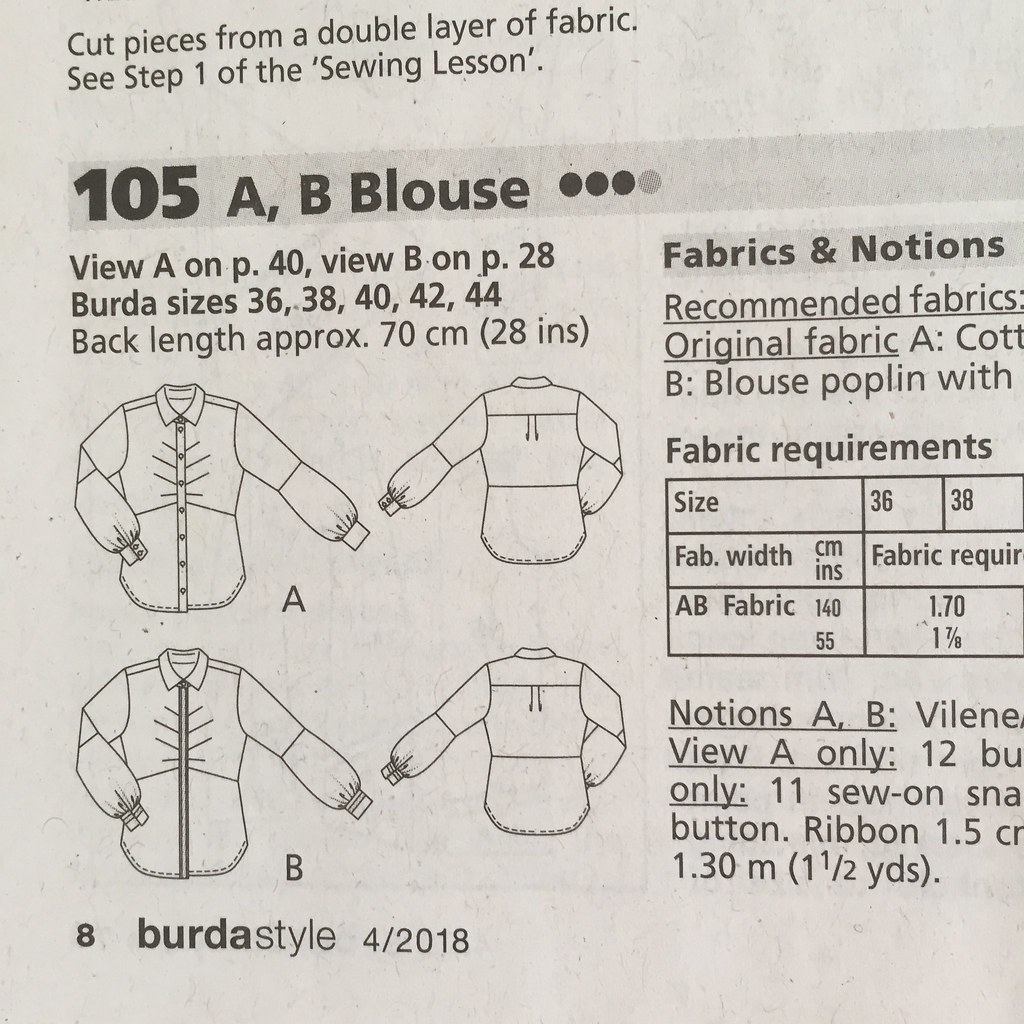This descriptive caption integrates details from all observations, with an emphasis on consistent and repeated elements:

The image depicts an instructional page from a sewing lesson on how to sew a blouse, rendered in black print on a white background with some grey accents. At the top left, the instruction “Cut pieces from a double layer of fabric. See step one of the sewing lesson,” is prominently displayed. Below this, a bold header reads "105A, B Blouse," followed by a row of three black dots and one grey dot. Below this header are diagrams showing both front and back views of two blouse styles, labeled A and B; blouse A features buttons down the front, while blouse B has a tunic style. 

Further down, small text directs readers to view A on page 40 and view B on page 28. It lists Burda sizes 36, 38, 40, 42, and 44, with a back length of approximately 70 centimeters (28 inches). At the bottom, the text reads “Burda Style,” and "Page 8 Berta style for 2008." 

To the right of the image, under the "Fabrics and Notions" header, recommended fabrics are specified: cotton for blouse A and poplin for blouse B. Fabric requirements are outlined in a rectangular box for sizes 36-38, alongside notes on fabric width and specific requirements for types A and B. Outside the box, additional notions needed are listed, including V-I-L-E-N-E, 12 buttons for view A, 11 sew-on snaps, and specific lengths for button ribbon (1.5 cm or 1.30 m, equivalent to one and a half yards). This comprehensive diagram serves as a visual guide for sewing the described blouses.